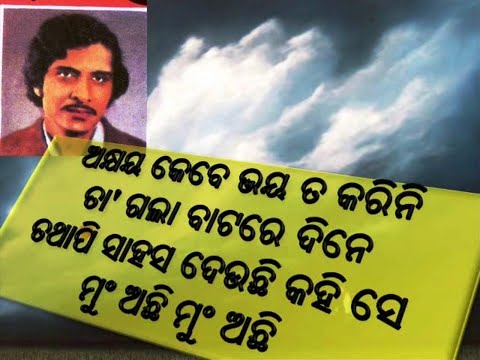The image is a complex collage consisting of three distinct elements. The background features a dark blue sky, interspersed with white, abstract clouds that give it a somewhat stormy appearance. At the bottom of the image, a sliver of green grass and a tree line can be seen. Superimposed in the upper left corner is a smaller photograph, reminiscent of a yearbook or ID photo. This smaller image depicts a man with dark wavy hair, an olive tan complexion, a mustache, and a slight beard. He is dressed in a brown or burgundy suit jacket paired with a white shirt, and his expression is serious, appearing mildly upset or indifferent. Above this composite image is a prominent, bright yellow rectangle featuring black text in a script resembling Sanskrit, the meaning of which is not understood by the viewer.